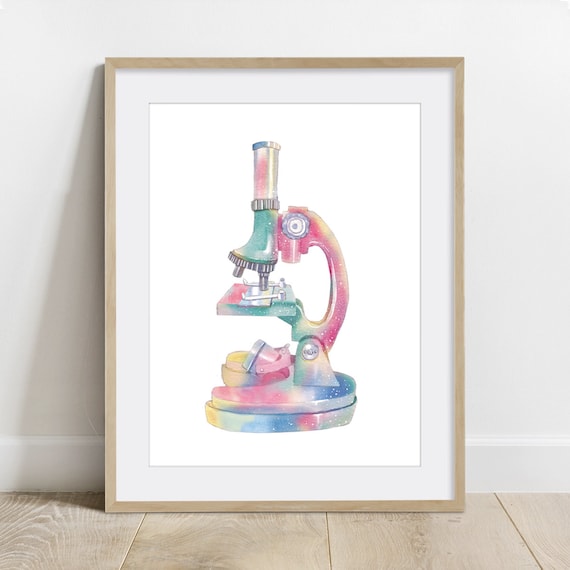The image features a framed illustration of a colorful, tie-dye rainbow-patterned microscope with muted shades of blue, red, yellow, and green. The detailed illustration showcases traditional microscope elements like the eyepiece, slide stage, and round base. It appears to be created using a combination of pencils and watercolors, all set against a stark white background. The rectangular frame has a light brown wooden finish and a white mat, and is leaning against a white wall with a grayish tint and a white baseboard. The whole setup rests on a light brown wooden floor, further emphasizing the vibrant colors of the art piece.